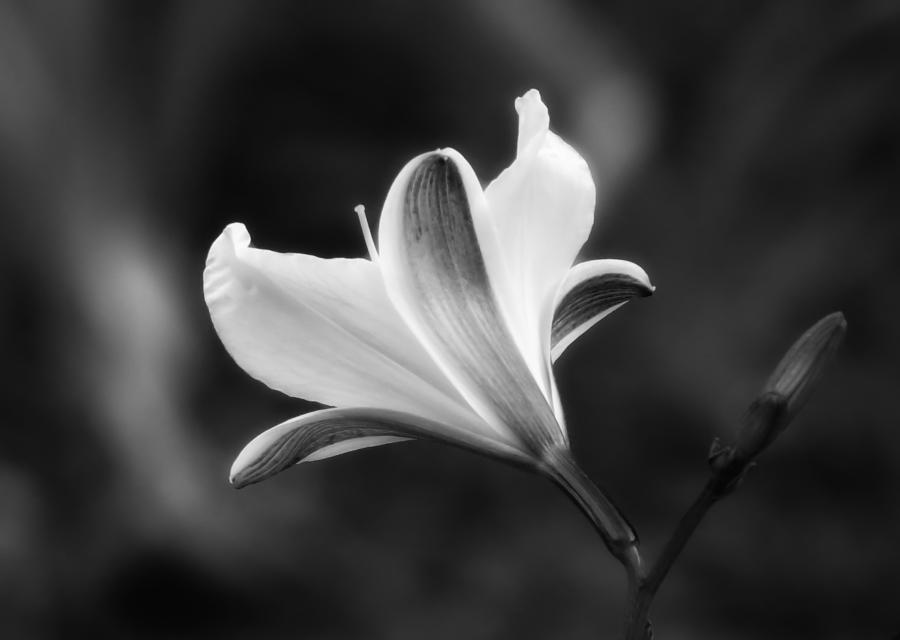This close-up black-and-white photograph captures the striking elegance of a lily in exquisite detail. The background is a dark, blurred expanse with white-to-gray streaks, providing a stark contrast that emphasizes the flower's delicate structure. Emerging from a deep, dark stem that rises from the bottom right of the frame, the main focus is the bloom of a single lily. The prominent flower bud, dark gray and oval-shaped, branches slightly up and to the right. Arcing up and to the left from a thicker stem section are the arching petals: dark underside petals extend leftwards and downward, another curves up to the right, and a final one arches towards the top of the frame. Nestled between these are two large white petals that fan out in small lobes, creating a glowing effect. A single white stamen prominently extends upwards from behind the central dark underside petal, contributing to the ethereal beauty of the image.